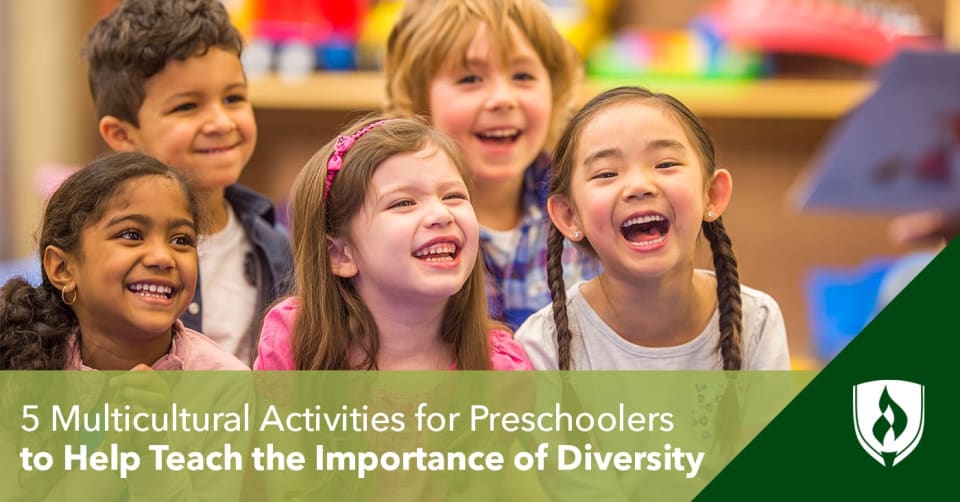The advertisement features a vibrant and joyful image of five children representing diverse backgrounds, all smiling and exuding happiness. Positioned in front of a colorful, blurry background likely filled with toys, these children include two boys and three girls of various ethnicities. In the back row, we see a Hispanic boy with dark curly hair, wearing a blue overall with a cross pattern of red and blue, standing next to a Caucasian boy with short blondish-red hair, who also sports a blue overall over a white shirt. In front, from left to right, there is a darker-skinned Hispanic girl with long hair draped over her shoulder, dressed in a light pink shirt; a Caucasian girl in the center with long brown hair, wearing a dark pink shirt; and an Asian girl on the far-right, with ponytails and pierced ears, wearing a white shirt. At the bottom of the image, a tan box contains white text that reads, "Five multicultural activities for preschoolers to help teach the importance of diversity." In the lower right corner, a green triangle encloses a white shield with a green design, serving as an emblem.